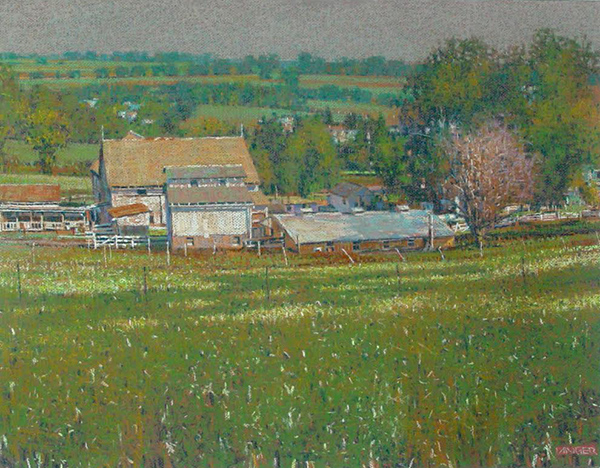This image is an intricately detailed painting of a rural farm property. In the foreground, a green landscape, accented with white specks and subtle hints of tan and beige, is prominently featured. A white gate on the left side leads into the expansive farm area. The property itself consists of several structures, dominated by a low one-story building, possibly a barn or house, which is notably long. Adjacent to this is a larger, over two-story barn with striking white walls and a reddish-gray roof. 

The natural surroundings include lush green trees and grass that frame the scene, blending seamlessly into the gray sky above. Scattered across the property, there are around five or six smaller buildings; some seem to function as stables or utility sheds, and one might even be a chicken coop. These structures vary in color, with the primary building painted white with a tan roof, others showcasing white or orange roofs, and yet another building displaying a yellow facade with a gray roof. 

The buildings appear constructed from stone and feature brick bases, contributing to their robust, utilitarian aesthetic. The entire landscape and structures are depicted in a rather muted, dull palette, employing lots of whites, grays, and lighter browns. Additional smaller buildings and trees populate the distant hillside, adding depth to the composition. The painting bears an illegible signature at the bottom right corner, although the last four letters appear to be "NGR." 

Overall, this artwork provides a serene yet detailed overview of a quintessential farmstead, where the natural and built environments coexist harmoniously.